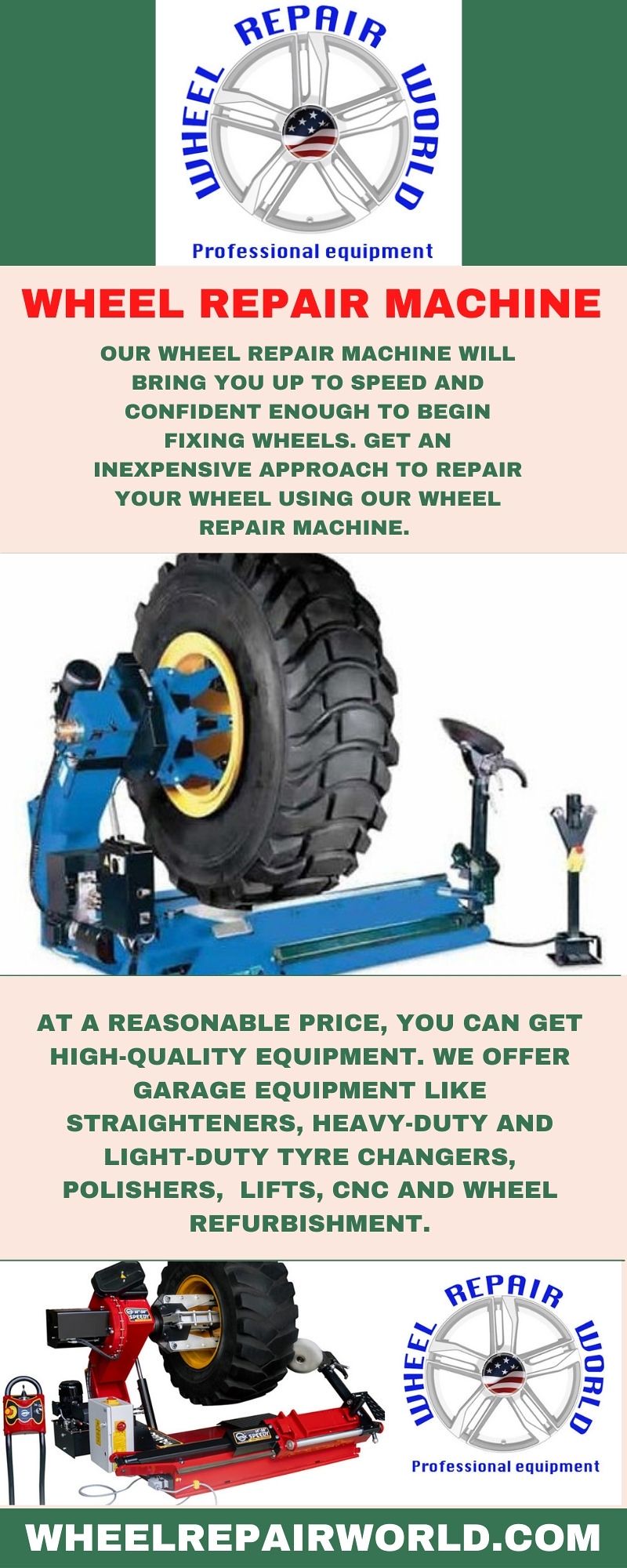The image is an advertisement for Wheel Repair World, showcasing their professional wheel repair equipment. The top part of the image features a green stripe, a white section with the Wheel Repair World logo, which includes an American flag and a wheel graphic. Blue text reads "Professional Equipment." Below, bold red text on a white background says "Wheel Repair Machine," followed by green text explaining that their machine will make you confident in fixing wheels affordably. The central part of the image displays a large wheel on a bright blue machine, accompanied by jack stands. Further down, green text highlights the reasonable price and high-quality garage equipment offered, such as wheel straighteners, tire changers, polishers, lifts, and CNC wheel refurbishment tools. At the bottom, there's a smaller red machine on the left side and the Wheel Repair World logo on the right, with the website WheelRepairWorld.com in white and green text.